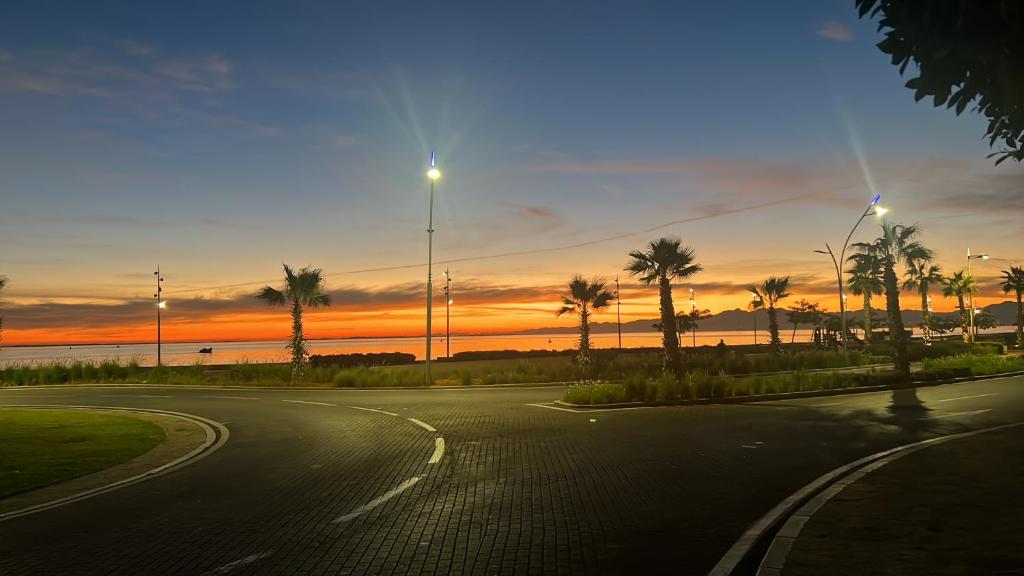This photograph showcases a dynamic scene of a cobblestone road stretching across the foreground. In the bottom right corner, a curved white line, resembling a half-circle, is distinctly visible. A similar half-circle is outlined in white on the lower left side of the image, adjacent to a patch of pavement which then transitions into lush green grass. To the right, an island filled with low green plants and stately palm trees acts as a median, separating lanes of traffic. The upper portion of the photograph reveals a breathtaking display of the sky, transitioning from a deep blue at the top to a lighter hue as it descends. This gradient culminates in a vibrant strip of bright orange and yellow, evocative of either dawn or dusk. Beneath this band of radiant color, the serene expanse of the ocean peeks into view, completing this picturesque setting.